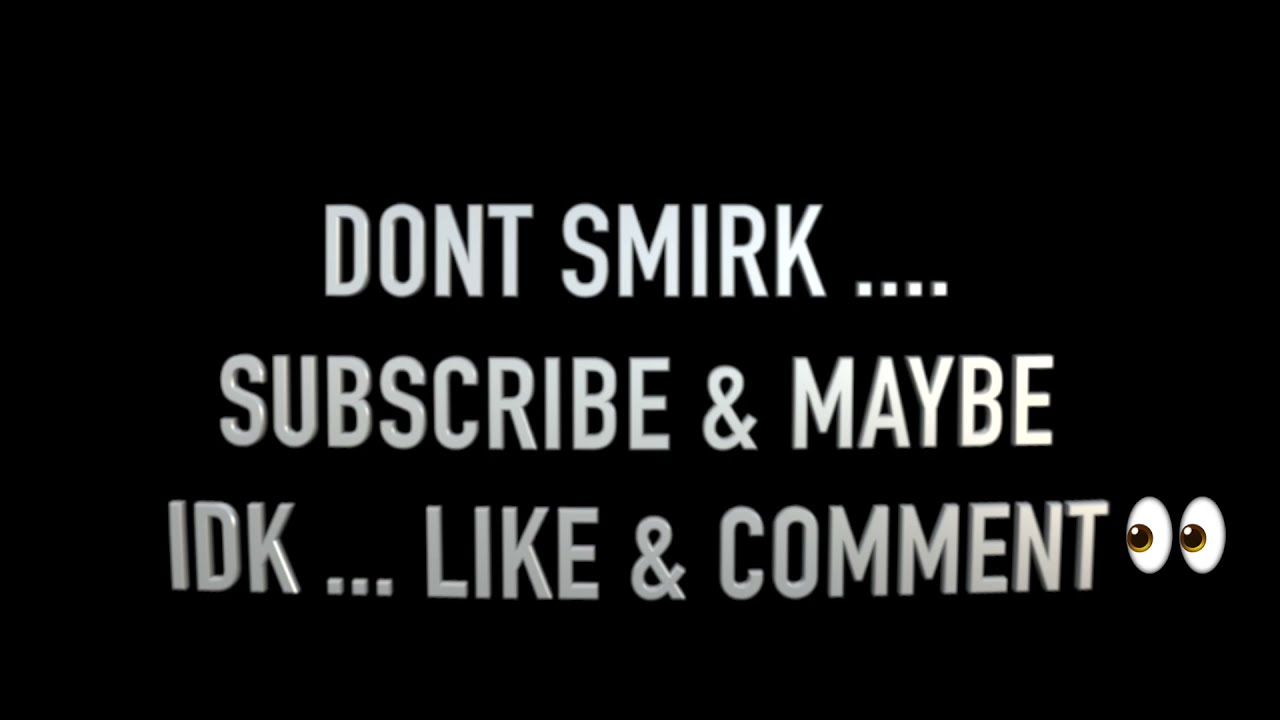This is a horizontally rectangular image with a solid black background. Centered in the middle, three lines of all-caps, blocky, light gray text are prominently displayed. The top line reads "DON'T SMIRK...." Noticeably, there is no apostrophe in "DON'T," and it is followed by an ellipsis consisting of four dots. The second line reads "SUBSCRIBE & MAYBE," with an ampersand used for "and." The third line lists "IDK... LIKE & COMMENT," where "IDK" stands for "I don't know." This line also includes an ellipsis composed of three dots and an ampersand for "and." To the right of the word "COMMENT," there are two disembodied white ovals with brown eyeballs outlined in gold, looking towards the text with a curious or suspicious expression. The composition is simple and stark, with no additional images or decorations.